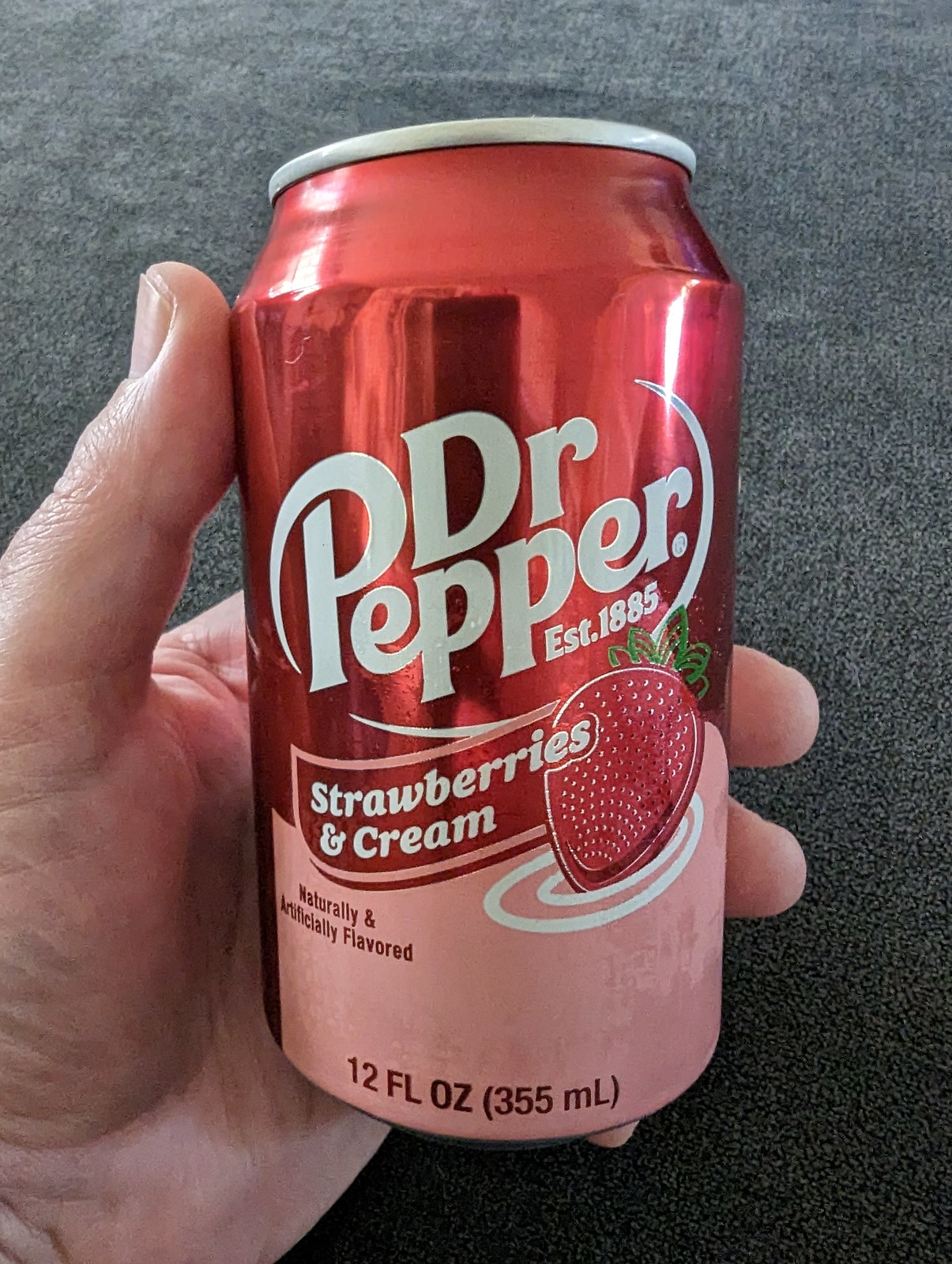The image is a high-quality, well-lit photograph, likely taken with a cell phone, showcasing a Dr. Pepper can in the new strawberries and cream flavor. The can is predominantly red at the top, transitioning to a pinkish hue towards the bottom. In large white letters, the label reads "Dr. Pepper EST 1885," with an additional white line typical of the brand's logo. Below, it states "strawberries and cream" in smaller white text, accompanied by a minimalistic illustration of a red strawberry with green leaves and white seeds. A delicate white swirl embellishes the area under the strawberry. Further down, the label mentions "naturally and artificially flavored" in red letters and indicates "12 fluid ounces (355 milliliters)." The can is being held by a white left hand, with the thumb prominently displayed along the side of the can. The background features a dark, almost black, soft surface, possibly a carpet or felt tabletop, adding contrast to the vibrant colors of the can.